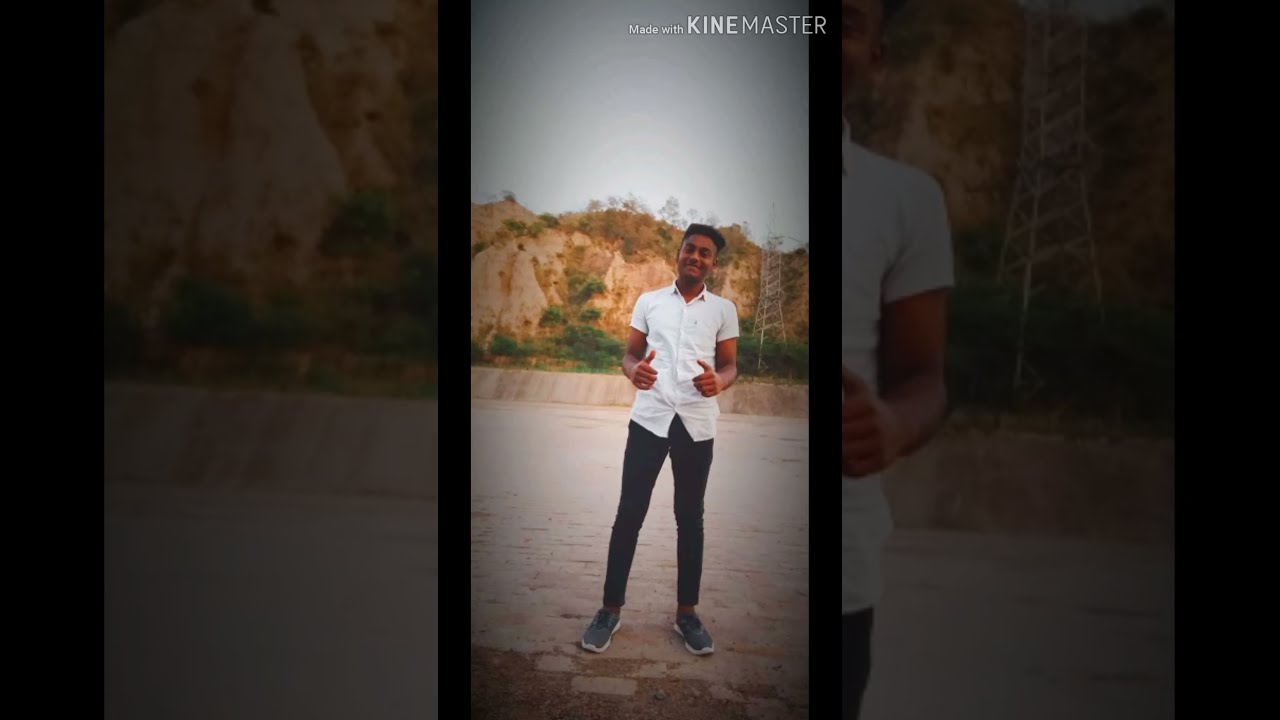This is a detailed descriptive caption of the picture:

A man with medium-dark skin, possibly of Indian descent, is standing in the middle of a wide stone or concrete area. He is wearing a white short-sleeved shirt, dark pants, and blue sneakers. The man, with short black hair, is smiling and holding both thumbs up in a pose reminiscent of Fonzie from "Happy Days." The backdrop features yellowish-tan cliffs with some green shrubbery, suggesting a desert-like environment that may be somewhere like Arizona. Further in the background, there is a metallic structure that could be a radio or cell tower. The image is set within a large, black letterboxed frame, where the vertical letterboxes on either side are nearly twice the width of the main portrait-mode image. At the top of this framed image, the text reads "Made with KineMaster."